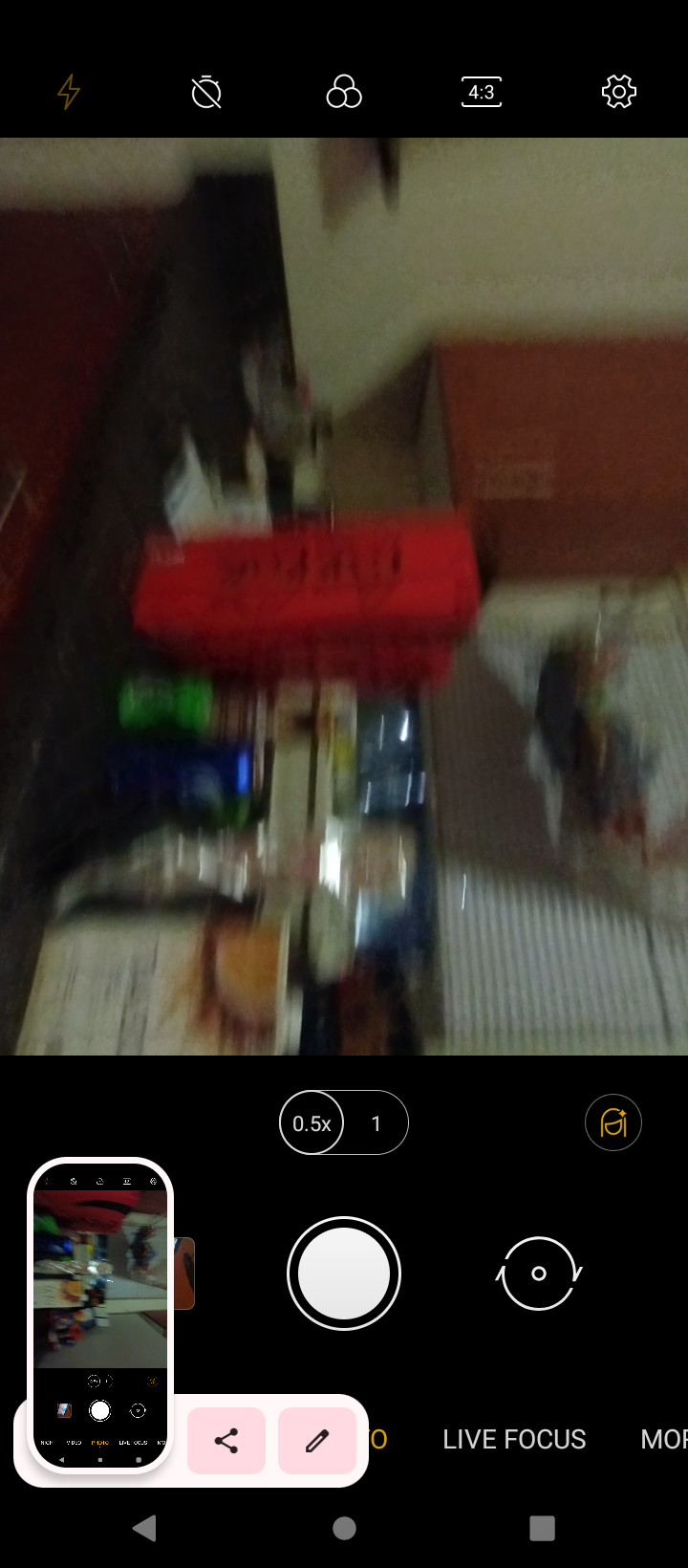This is a screenshot taken from a phone's camera application, showcasing the interface and on-screen icons. The top and bottom of the screen are bordered by black bars containing various icons. In the top left corner, there is an orange lightning bolt icon representing the flash setting. Beside it to the right, a white icon resembling a circle with a dash through it indicates a specific camera mode. Adjacent to this is an icon consisting of three stacked white circles, possibly denoting filter or effects options. Following is a rectangular icon labeled "4:3," indicating the aspect ratio of the photo. To the far right on the top bar, there is a white cog icon, likely representing settings.

At the bottom center of the screen, a large white circle serves as the shutter button, surrounded by a white outline. To its right is an icon showing two arrows forming a circle, used for switching between the front and rear cameras. In between these interface elements, the camera viewfinder shows a blurred image consisting of various objects scattered on a floor. Notable amongst these objects is a red box of soda cans. Other indistinct items reflect faint light, further adding to the cluttered scene.